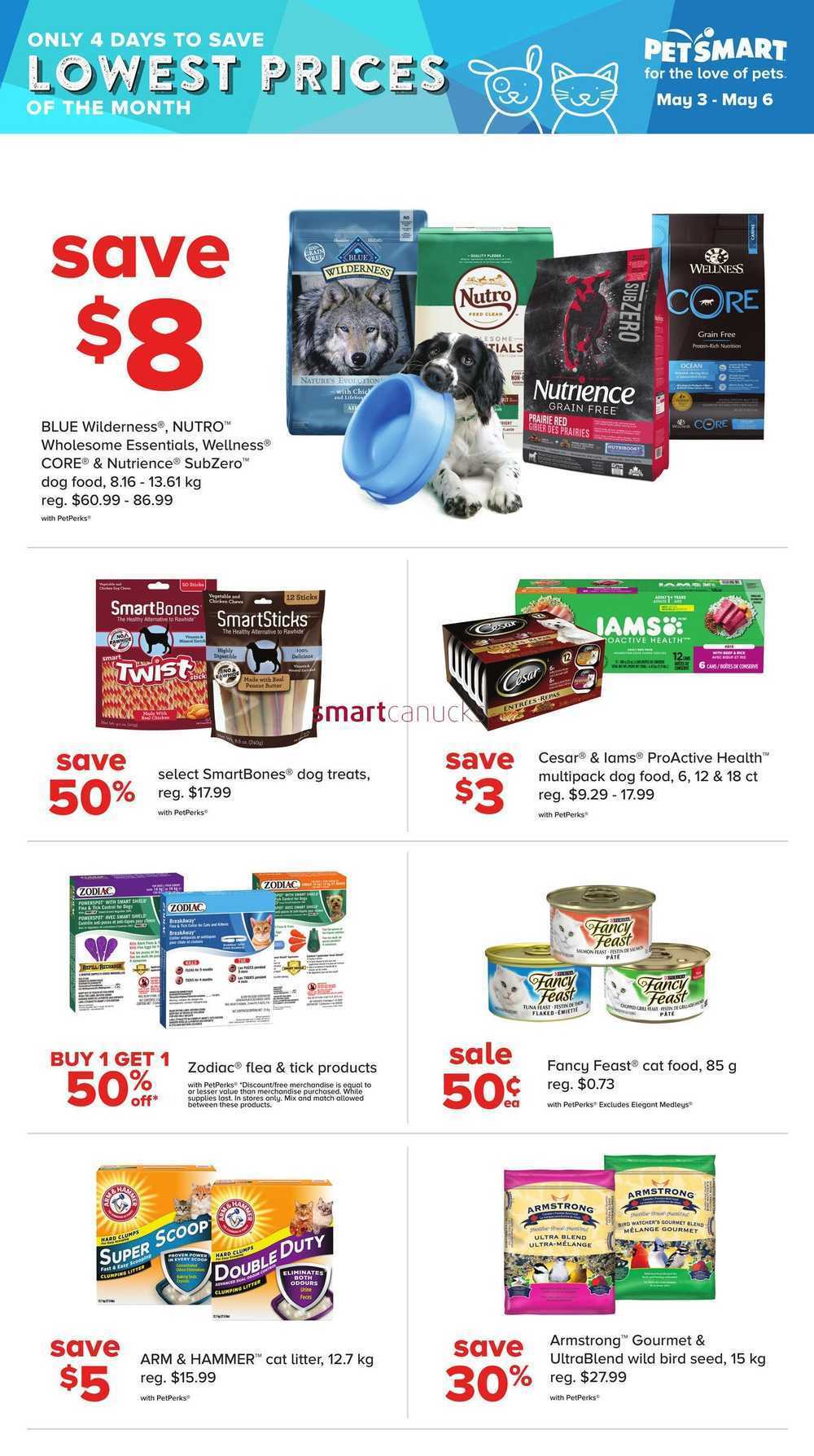The promotional image from PetSmart features a prominent blue banner at the top, stating "Only Four Days to Save: Lowest Prices of the Month" and highlighting the sale period from May 3rd to May 6th. Below this, on a crisp white background, are various pet products with corresponding discounts.

Centered prominently is a charming puppy holding a blue dog food bowl in its mouth, surrounded by four different bags of dog food brands. Accompanying text announces a discount of $8 on Blue Wilderness, Nutro, and Wholesome Essentials dog food, although the details are slightly blurred.

Below the dog food section are two bags of dog treats with a bold "Save 50%" offer on SmartBones. Adjacent to this, an IM food product boasts a $3 discount.

On the left side of the lower section, there are three boxes of cat litter, advertised with a "Buy One Get One 50% Off" deal. To the right, three cans of Fancy Feast cat food are showcased with a listed price of just 50 cents each.